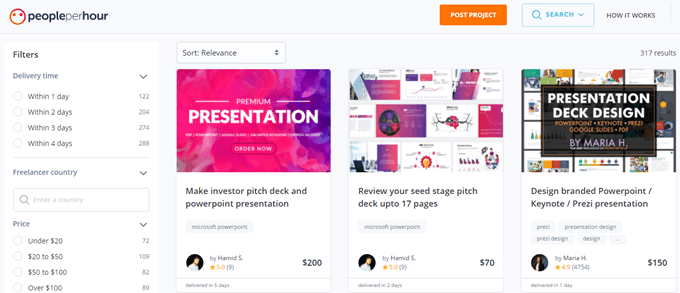This cropped screenshot captures the detailed layout of the People Per Hour desktop web page. At the top, the header is presented in a light gray color. On the far left of the header, there is the People Per Hour logo, featuring a red smiley face icon followed by the text "people per hour" in lowercase letters. To the right of the logo, there are two distinct boxes. The first box, which is orange, displays the text "Post Project" in small white font. Adjacent to it is a search box with a blue outline and blue text, accompanied by a dropdown menu for search categories. Further to the right, "How It Works" is written in small black letters.

Below the header, on the left side, there is a vertical panel containing various categories. At the top in small bold black font, it says "Filters." Directly beneath, the category "Delivery Time" is listed in small blue letters, and it is expanded to show different delivery options with corresponding numbers of available freelancers. Specifically, it lists:
- "Within 1 day" with 122 freelancers
- "Within 2 days" with 254 freelancers
- "Within 4 days" total

Following the "Delivery Time" section is the "Freelancer Country" category, which is not expanded. Below that is the "Price" category, which shows a vertical list of prices along with the number of freelancers available for each price point.

On the main section of the page, there are three prominent thumbnails displayed within large boxes. Each box features:
1. A photo at the top, followed by a brief description
2. The freelancer's name, their rating, and their cost

The first box advertises "Premium Presentation" with a background of purple and pink smoke. Beneath this visual, the description reads "Make Investor Pitch Deck and PowerPoint Presentation." The freelancer boasts a 5.0-star rating based on 9 reviews, and the service is priced at $200.